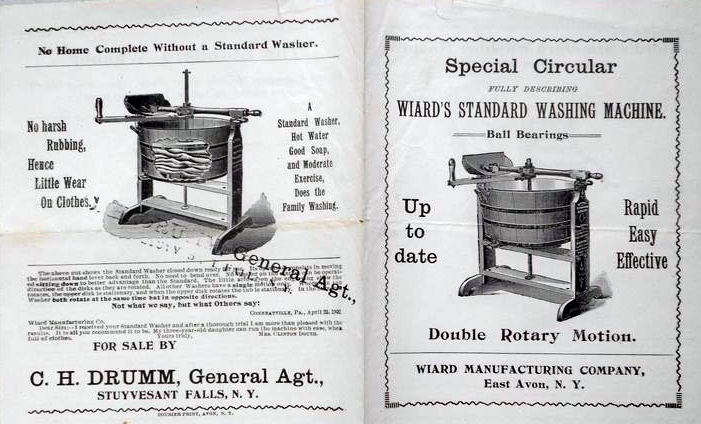The image depicts a pair of vintage advertisements from an old magazine or newspaper, displaying the front and back cover of a pamphlet or a full-page spread. Both ads showcase an early 20th-century washing machine crafted with a wooden tub and a metal interior, resembling a wide barrel with a crank mechanism on top, operated manually without electricity. The advertisement on the right, titled "Special Circular," promotes "Wyard's Standard Washing Machine," emphasizing its "up-to-date, rapid, easy, effective, double rotary motion," and credits its manufacture to Wyard Manufacturing Company, East Avon, New York. The image on the left features the same washing machine, with a transparent illustration of the tub revealing clothes inside, accompanied by the tagline, "No home complete without a standard washer. No harsh rubbing, hence little wear on clothes." The ad concludes with, "Hot water, good soap, and moderate exercise does the family washing," and states it's sold by C.H. Drum, General Agent, Stuyvesant Falls, New York. Though somewhat blurry, a date on the image appears to say "April," possibly from the year 1932 or 1922.